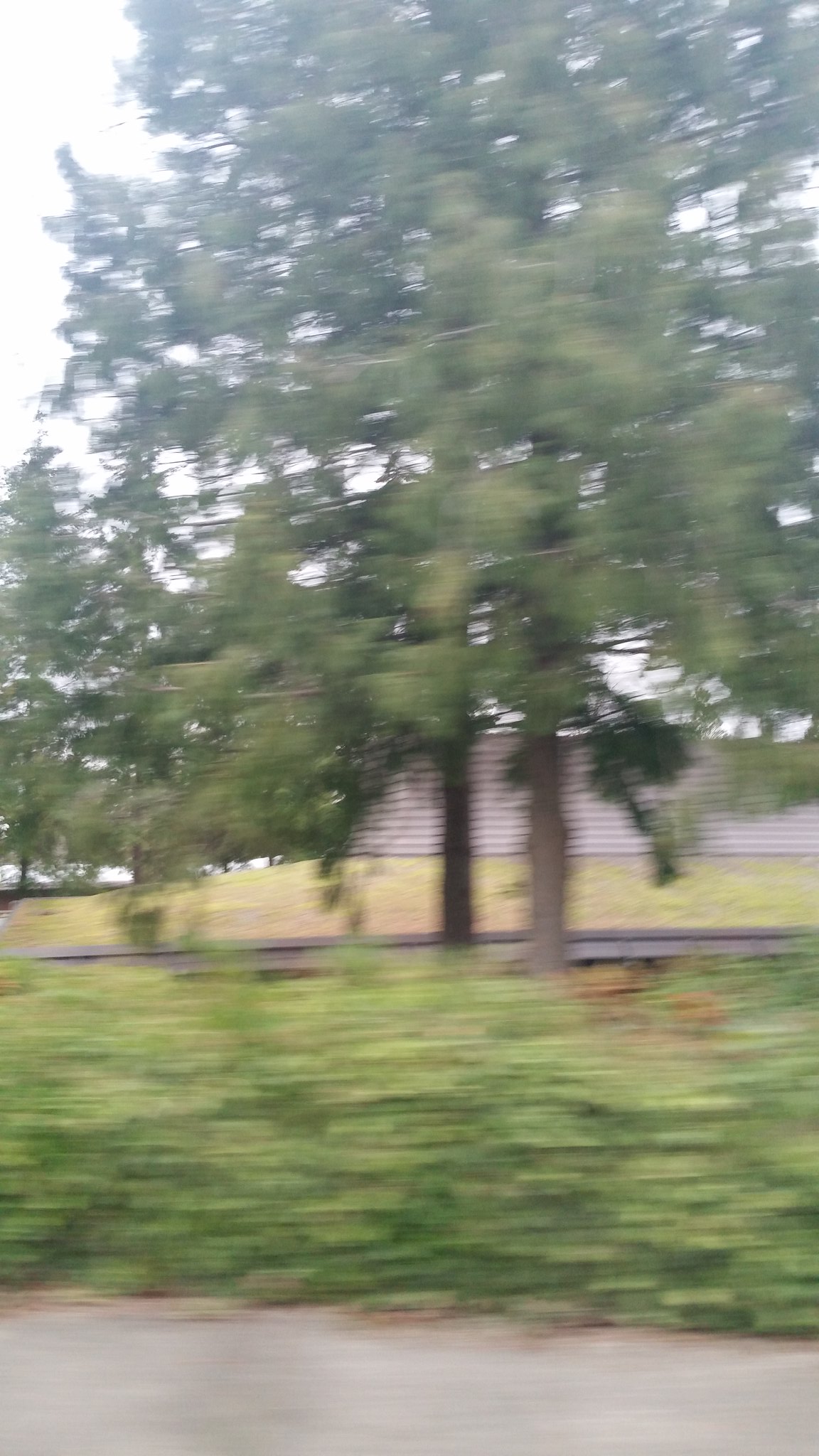In the foreground of this outdoor photograph, two tall trees frame a walking path, their trunks clearly visible but their branches extending out of the shot from the top and right-hand side. The bright, almost white sky forms the distant background, emphasizing the height and prominence of the trees. Between them, the paved path leads the eye towards a green area where well-manicured grass and a small, white building are discernible. Flanking the path in the immediate foreground is a grassy area, reminiscent of a park setting, with hints of an additional path or roadway intersecting the scene. Though the image is slightly out of focus, the composition captures a tranquil yet dynamic outdoor environment.